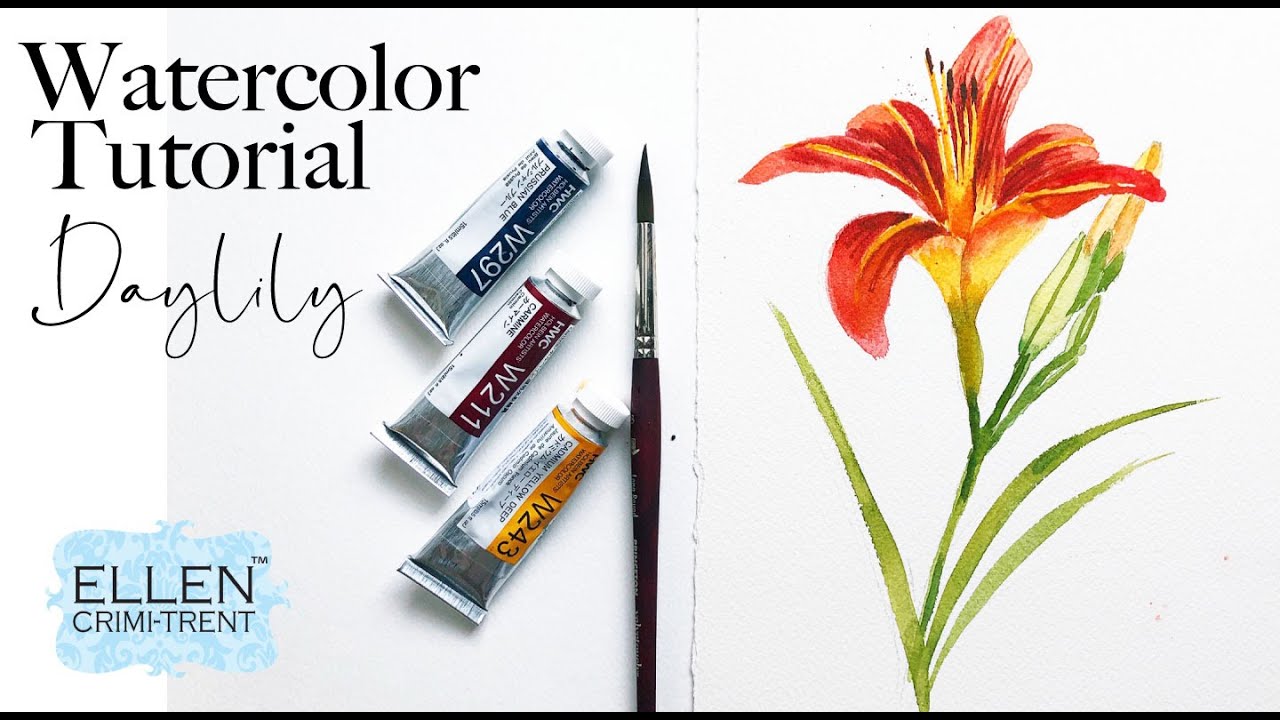This is an illustrative poster promoting a watercolor tutorial on painting a daylily by Ellen Crimmy-Trent. The design is split in two sections against a solid white background, framed by black lines at the top and bottom. In the center, a paintbrush with a brown handle stands upright, dividing the image. 

On the left side, three tubes of watercolor paint are displayed next to the title "Daylily." The paints are labeled with codes: blue (W297), maroon (W211), and yellow (W243). In the left corner, a splash of blue features the artist's name, Ellen Crimmy-Trent, in black lettering.

The right side showcases the tutorial's subject, a vividly detailed daylily. The daylily is depicted with a green stem and leaves, transitioning into bright yellow at the base of the bloom. The red petals are accented with yellow lines, and the flower's center features prominent yellow stamens. This composition highlights the vibrant colors achieved with the specified paints, providing a clear and detailed visual guide for the tutorial.